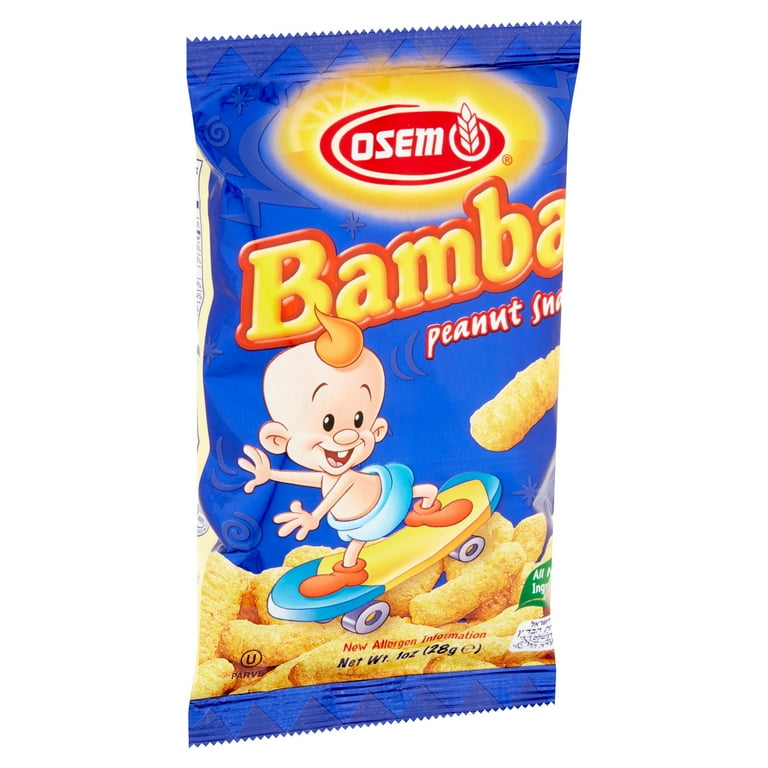This image features a vibrant, electric blue bag of Bamba peanut snacks. Prominently displayed at the top of the bag is a yellow oblong shape enclosing a red oblong with white writing that reads "Osem," accompanied by a white leaf logo. Below this logo, the word "Bamba" is written in bold yellow text with a red outline, followed by "peanut snacks." The bag showcases a cartoon baby with a lightly tufted sprig of hair in the center of his bald head. The baby, dressed in blue shorts and orange shoes, is smiling and looking backward while riding a yellow skateboard with blue ends and wheels. The baby is depicted skateboarding over the peanut snacks, giving a playful impression. Additional details like the allergen information and net weight (1 ounce, or 28 grams) are prominently displayed at the bottom of the bag.